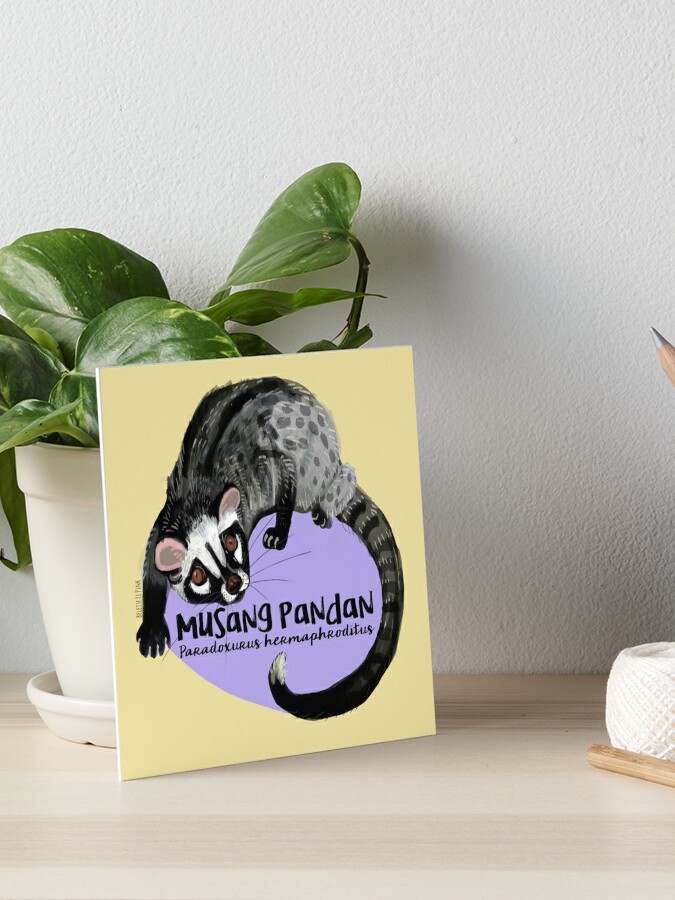The image depicts a small painting propped against a large white ceramic pot with a green plant featuring shiny, large, semi-pointed leaves. The scene is set on a wooden table, and the wall behind features a subtle pattern. To the right of the painting, there is some white twine, a brown stick, and the point of a pen. The artwork itself, standing out with its pastel colors, has a light yellow background and showcases a gray possum-like animal, called a "Mu Sang Pandan," with pink ears, a white-tipped long tail, and a face patterned in white and black with brown eyes and nose. The creature is curled around a purple, egg-shaped form. Beneath the possum's name, there's an illegible cursive text. Additional subtle hues of green, white, and brown are scattered throughout the scene to complement the composition.